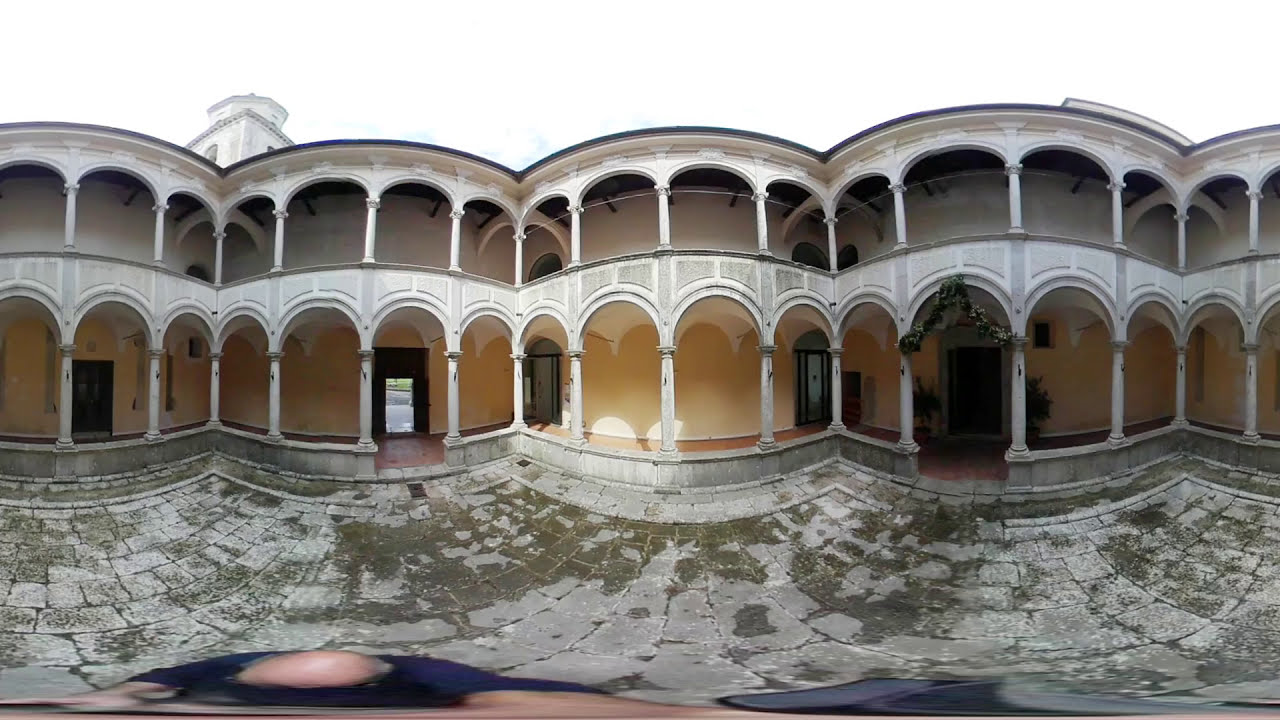This 360-degree panoramic image shows the courtyard of a two-storied building, presenting an intricate and detailed view. The courtyard features weathered, grayish-black stone ground that seamlessly integrates with the white and grayish-white stone archways supported by matching columns. These archways create a rhythmic pattern around the courtyard, giving a sense of historic charm. The building itself has a yellow lower story and a white upper story, framed by arches on both levels. A red cobblestone path leads to the building, diverging through openings in the courtyard walls.

In the top left corner of the image, a taller, square-shaped white stone building with a black roof is visible in the background, adding an extra layer of depth. An elaborate front porch with white awnings and columns suggests this might be either a home or a hotel. The second level of the porch mirrors the first, with more arches creating a covered space. A small tower emerges on the left, though it’s not clear if it belongs to this building or another nearby structure. 

A person is capturing this scenic view with a camera on a selfie stick, their bald head and blue shirt slightly visible. The panoramic stitching skews the usual perspective, aligning all four walls in one continuous, horizontally aligned rectangle, resulting in a cool effect where the entire courtyard and its architectural details are laid out in a single, cohesive image.